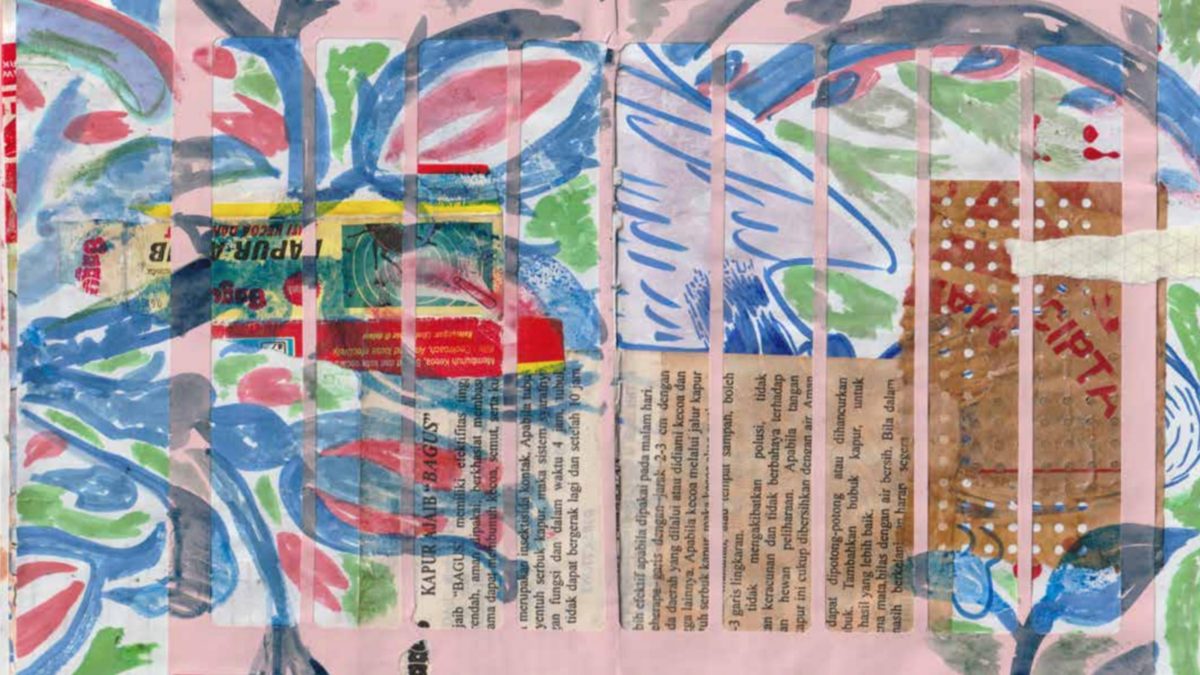This highly detailed abstract collage art piece combines vertical strips of decorative paper, all placed on a pink background. On the left side of the image, a wide strip dominates, featuring intricate watercolor designs in blues, reds, and greens, which resemble feathery patterns and floral motifs akin to a peacock's plumage. Nine equally sized strips filled with similar evocative, vibrant designs follow in the middle. The right side of the collage is marked by a thin strip, complementing the central theme.

Interspersed within these colorful patterns are segments of newspaper print and book clippings, oriented sideways and containing text in various foreign languages, adding a layer of cultural intrigue. Noticeably, the lower half of some strips include this undecipherable text. The collage displays prominent colors—blue, green, and red dominate, creating a busy, dynamic scene.

Additional elements enhance the complexity: the bottom right corner features a blue leaf, whilst on the right side of the composition, there are abstract shapes resembling bird wings and a piece of brown paper bag with visible punched holes and lettering spelling out "SIPTA." This confluence of materials and colors renders the collage vibrant and visually engaging.